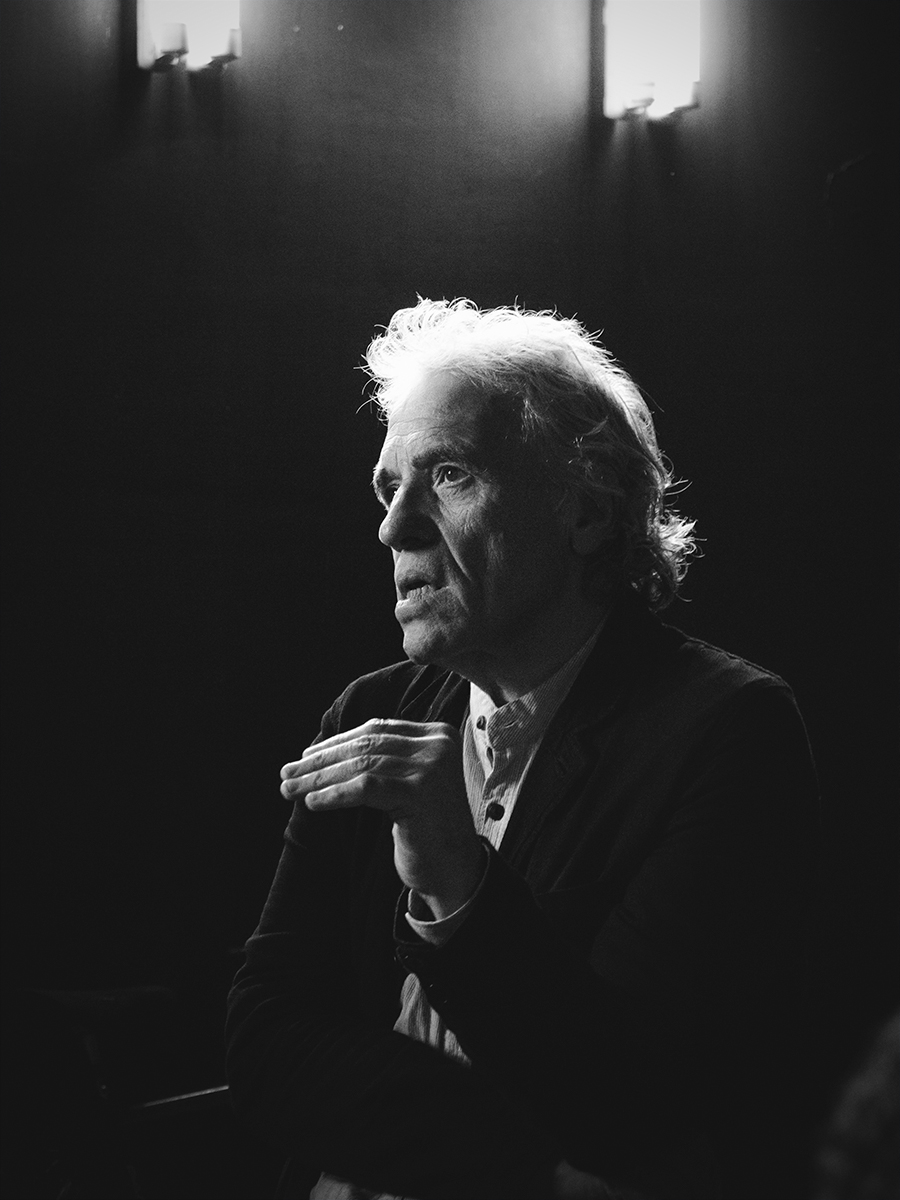In this dramatically lit, black and white photograph, we see an elderly man seated in a chair positioned centrally against a dark, dimly lit background, likely indoors. The image highlights only shades of black, white, and gray, creating a somber atmosphere. The man, who appears very old and thin with loose skin, is facing to the left, slightly hunched over. He has sparse, light-colored hair that reflects the few light sources positioned at the top of the image, giving his hair a white glow. He is wearing a dark jacket over a lighter-colored shirt. His left arm is bent at the elbow with his fingers drawn together and bent downwards at a 90-degree angle, while his right hand rests across his belly. His mouth is slightly open, revealing the bottom row of his teeth. The stark contrasts between the highlighted features of his face, hair, and fingers against the predominantly dark setting enhance the dramatic, almost haunting, quality of this photograph.